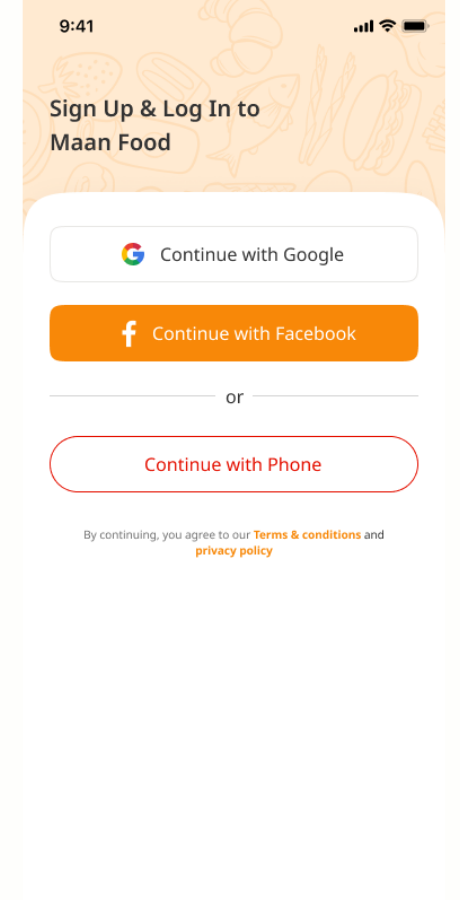Screenshot of a cell phone screen displaying the login page for the Mon Food app. The time is prominently shown in bold black font at the upper left-hand corner, reading "9:41." To the upper right, icons for cell phone reception, Wi-Fi signal, and battery status are visible. The screenshot is suffused with a light tan, almost orange hue at the top, creating a gradient background.

Amidst this light background, several images blend in, including a chestnut, a fish, a hamburger, and what appear to be two straws. A vivid picture of a strawberry is also visible. On the left side of this gradient area, "Sign Up and Log into Mon Food" is written in bold black text. Below this section, the background shifts to white, featuring a series of buttons for login options: "Continue with Google," "Continue with Facebook," and "Continue with Phone," separated by the word "or." This portion clearly represents the login screen for the Mon Food application.